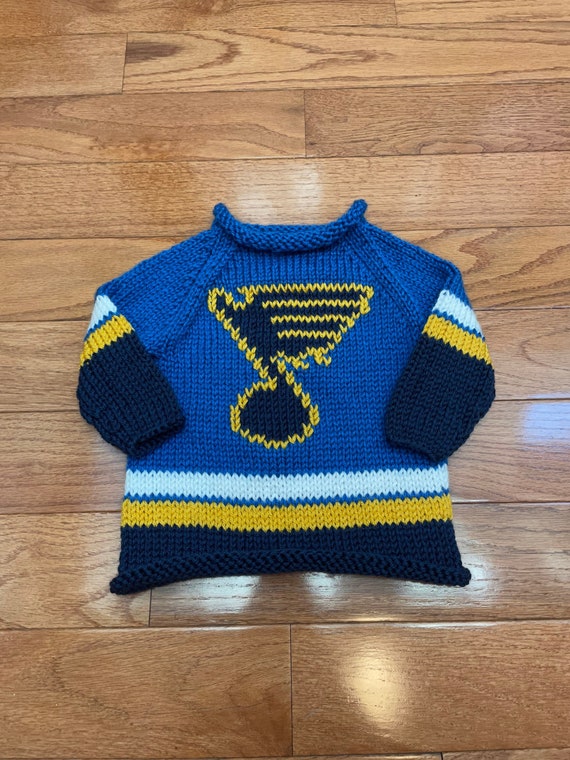This image features a very small, hand-knitted Philadelphia Flyers jersey, likely created for a baby, dog, or as a novelty item like a beer cozy. The jersey is centrally placed on a shiny hardwood table and photographed from a top-down perspective, most likely with a phone camera. The primarily blue jersey showcases the Philadelphia Flyers logo prominently in the center, encircled by a black figure outlined in yellow that resembles a musical crotchet with wings. Both sleeves and the bottom hem of the jersey feature coordinated stripes: a white stripe followed by a yellow stripe and ending with a navy blue stripe. The intricate details and vibrant colors make this knitted jersey a charming and visually appealing piece.